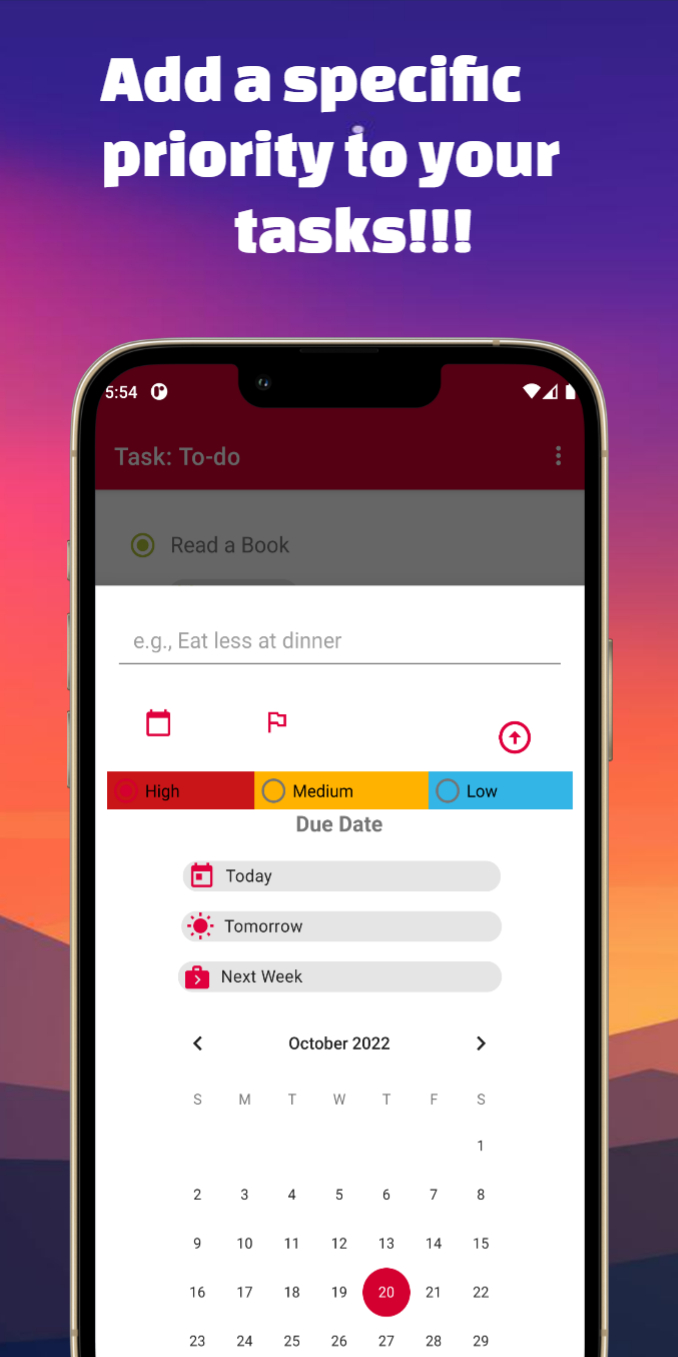In the image, the chat interface features a rainbow of colors, transitioning from blue to purple, then to red, purple again, and finally black. A smartphone screen displays a variety of notifications and statuses: the time reads 5:54, the WiFi signal is noted as full but showing no actual connection, and the battery icon indicates a full charge. Among the notifications, there's a prompt to "read a book," another suggesting to "eat less at dinner" signed by "Condor," and a flag positioned at the top. The flag seems to indicate priorities: orange signifies medium importance, blue denotes low importance. A due date schedule lists tasks and their deadlines, categorizing them as today, tomorrow, and next week. Additionally, the timeline reflects a series of dates ranging from October 2022 to specific days labeled from Sunday to Saturday, numerically spanning from 1 to 20.